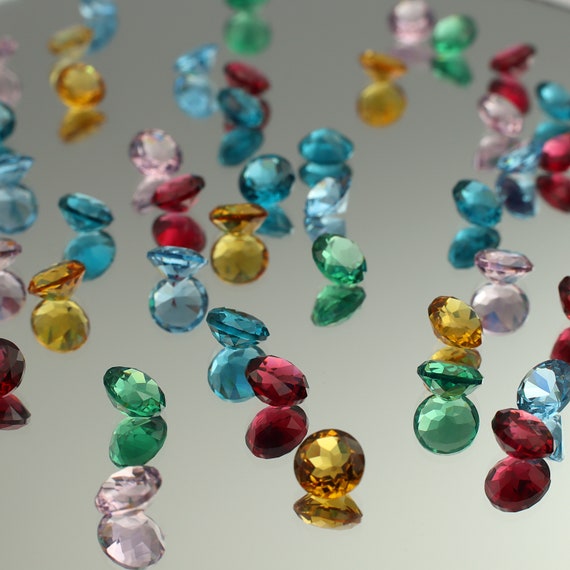The image features a collection of variously colored gemstones—green, blue, yellow, red, light pink, light purple, and turquoise—scattered across a reflective surface that appears to be a mirror. The light gray background sets a neutral stage, enhancing the vibrant hues of the gemstones. Each jewel is cut with multiple facets, resembling the shape of a diamond, and they are all positioned on their edges, causing the mirror to reflect their intricate forms and vivid colors underneath, almost as if showing a duplicate set beneath them. The light subtly interacts with the gems, highlighting some while leaving others in softer tones. The arrangement and reflections give an impression of an opened jewelry box or clamshell, adding to the overall artistic and elegant feel of the scene.